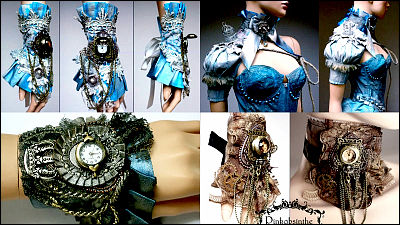This image is an elaborate collage featuring eight individual photos of steampunk-inspired fashion accessories. The top row comprises three close-ups of a woman's hand adorned in an ornate blue glove with finger holes, accentuating intricate lace and embellishments. To the right, two images reveal the upper body of a woman dressed in a matching denim-blue, velvet bustier adorned with ornate accents and a delicate tie around the neck, her face turned slightly to her left. In the middle row, the left image depicts another detailed shot of a woman's hand facing eastward, showcasing an elegant golden watch wrapped with fabric and ruffled lace trim. In the lower right, two images display brown gloves with gold accents and finger holes, emphasizing their vintage steampunk aesthetic. The lower-center part of the image features "pinkosynth tea," presumably the watermark.